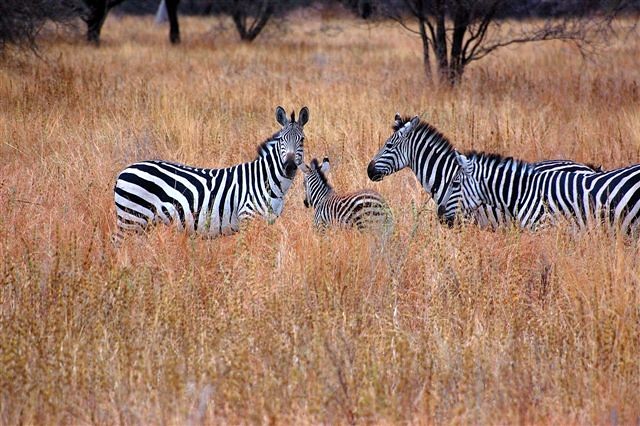In the photograph, a picturesque grasslands scene unfolds with four zebras standing amidst a dense sea of tall, brownish-yellow grass. We see a trio of adult zebras accompanied by a smaller baby zebra centrally positioned among them. The zebras' striking black-and-white patterns stand out sharply against the muted backdrop of the grasslands. 

On the left, one zebra faces the camera directly, its body angled slightly left while its head is turned right, creating a captivating gaze towards the viewer. This zebra stands out prominently due to its attentive stance. Adjacent to this zebra, the baby zebra is facing away, showing its back to the camera. Behind the baby, another adult zebra is oriented to the left, its side profile clear, and seamlessly blending with yet another zebra, also facing left, whose presence is subtly interwoven with the surroundings. 

In the background, several trees rise from the horizon, bare branches hinting at a fall setting. Some cut-off tree branches are visible in the foreground, adding a natural frame to the scene. The overall tableau not only highlights the zebras’ natural beauty and social arrangement but also the rich texture of the environment they inhabit.